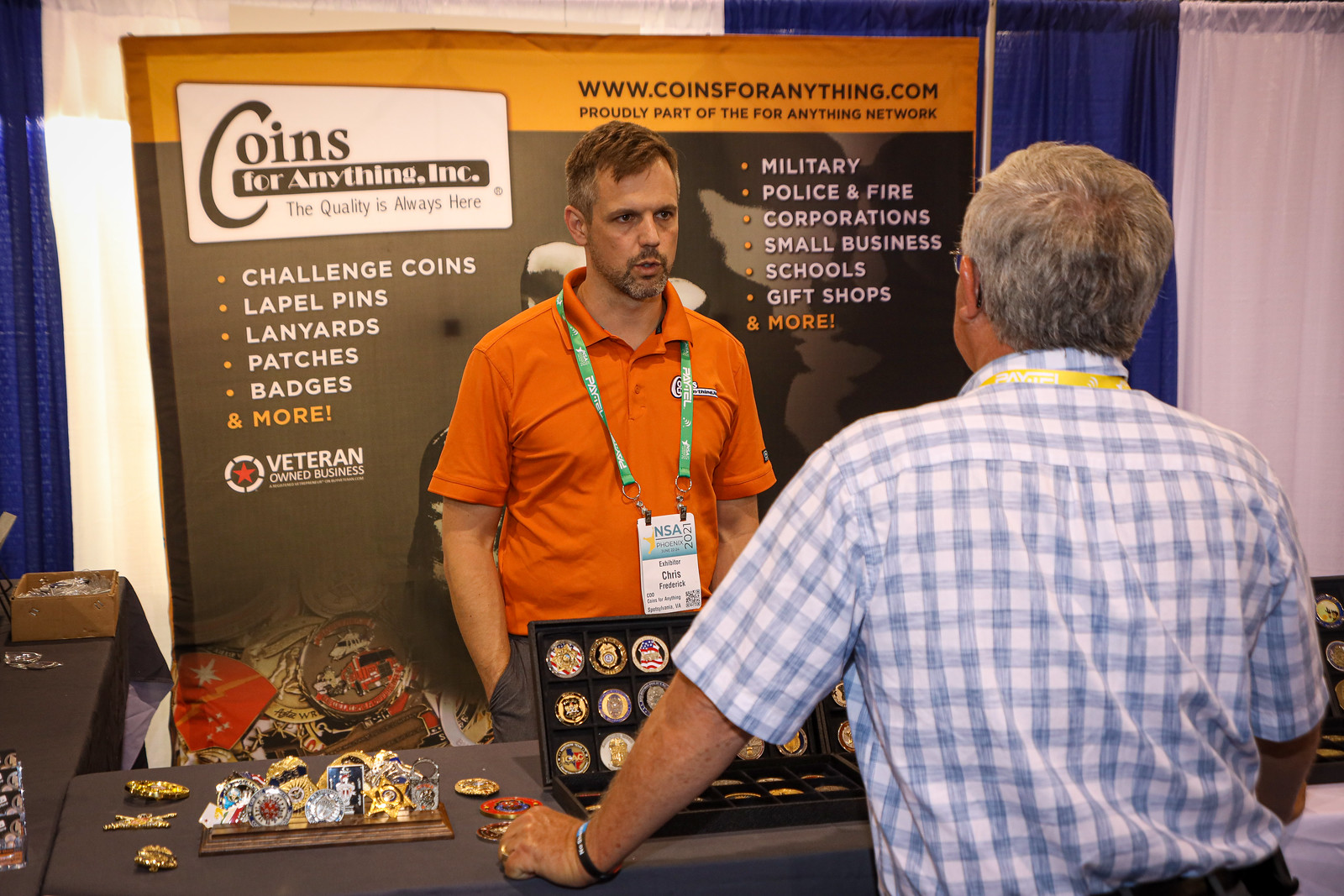In the photograph, two men engage in conversation at a booth featuring a display of various collectibles. The man behind the table, wearing an orange polo shirt and a lanyard, stands in front of a prominent banner for "Coins for Anything Inc." The banner, which highlights the company's offerings such as challenge coins, lapel pins, lanyards, patches, badges, and more, reads "The quality is always here" and denotes the business as veteran-owned. The banner also includes a website address, coinsforanything.com, suggesting it is part of the For Anything Network, and lists potential customers like military, police, fire corporations, small businesses, schools, and gift shops. 

In front of the man lies a brown tablecloth-covered table with an array of shiny objects resembling sheriff's badges, patches, and possibly belt buckles. The man he is speaking with has his back to the camera and is dressed in a blue and white checked shirt paired with a yellow lanyard. They both appear to be discussing the items on display, which range from coins to various memorabilia, indicating a typical exchange at an event or trade show booth.